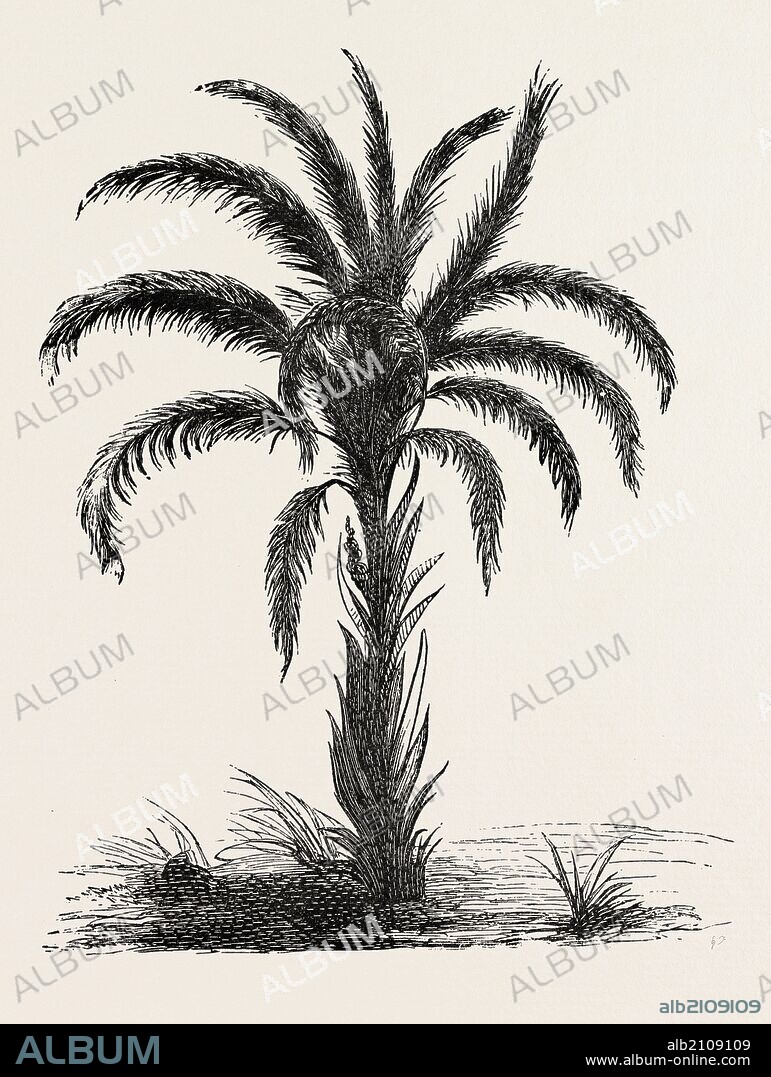This is a detailed drawing of a palm tree, rendered in black ink with fine lines on a slightly textured, off-white paper. The tree features drooping, spiked leaves that extend outward from both the top and along the entire length of the trunk, which is atypical for traditional palm trees. The illustration includes various scribbles of plant life on the ground surface beneath the tree. This artwork, with its intricate pen lines, appears to be a high-quality stock illustration, marked with several watermarks that say "ALBUM" in various colors and an opaque overlay across the image. Additionally, "ALBUM" appears in blue in the lower left corner along with the text ALB2109109 and the website www.album-online.com, written twice—once at the bottom and once in blue.